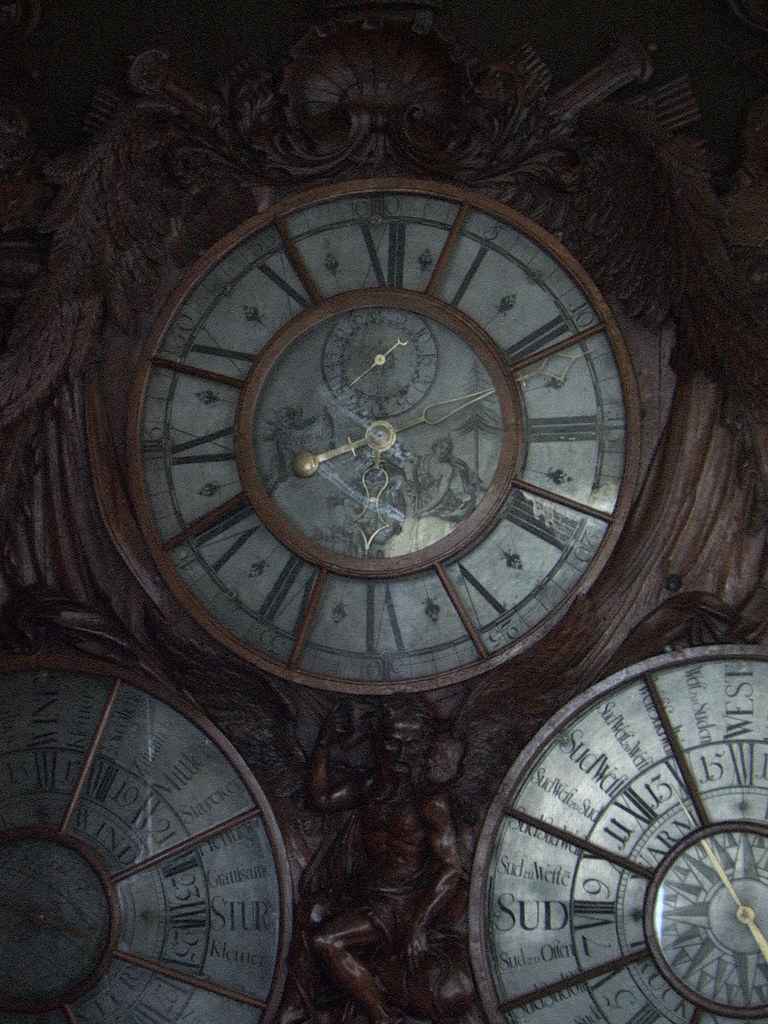This image captures a mesmerizing scene of three elaborate clock-like devices viewed from beneath, possibly taken from the vantage point of someone standing under an atrium. The clocks feature a distinctive bronze finish, with intricate metal or pewter detailing. 

The topmost timepiece, devoid of traditional numbers, uses unique symbols to denote the passage of time. It features a secondary inner circle with a miniature clock face, adding to its complexity. The two lower devices appear to serve a different function, potentially displaying dates, as they are adorned with script in a foreign language and the word "West" is discernible. These clocks also incorporate numerical and compass elements into their design, suggesting navigational or timekeeping functions.

Adding to the ornate presentation are intricate carved creatures positioned between the clocks, enhancing the overall aesthetic and lending a sense of artistry and craftsmanship to the entire ensemble.